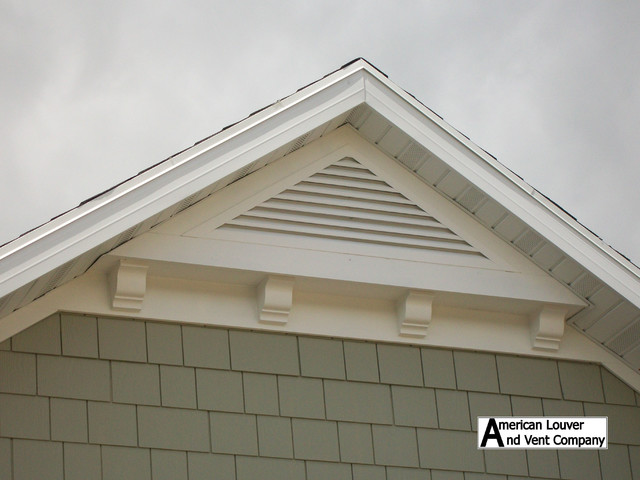This photograph captures the peak of a house adorned with architectural details and under ominous skies. Dominating the center is a large, triangular-shaped vent painted in a warm cream color, prominently displaying the label "American Louver and Vent Company" at the base of the image. The louvers of the vent run horizontally, adding a distinct texture to the triangle's peak. Beneath this vent, there are decorative braces that support it and extend outward, adding to the visual interest. The house's exterior features cedar siding shingles in a greenish-gray hue, arranged neatly in horizontal lines. Above, the dark gray shingles cover the roof, juxtaposed against white eaves. The sky overhead is filled with dark gray clouds mingled with patches of white, creating a moody atmosphere devoid of any visible blue sky.